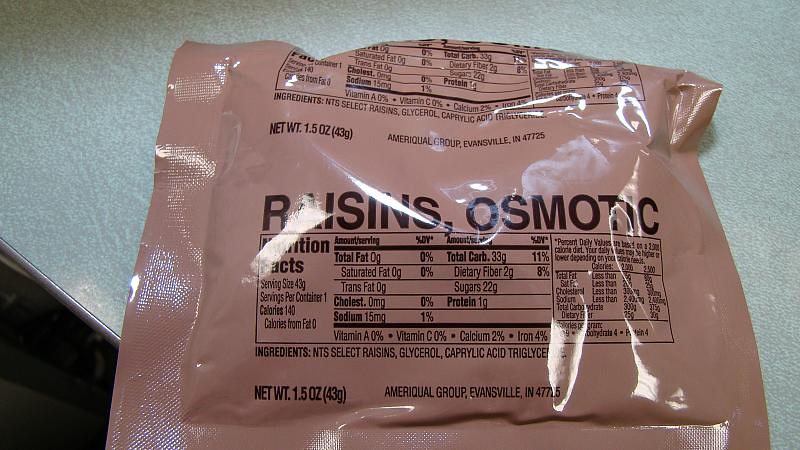This close-up photograph captures an MRE (Meal Ready to Eat) package, prominently displayed against a gray marble countertop speckled with white. The surface and the MRE both reflect light from white overhead lighting, enhancing the texture and details. The MRE package, a dark chocolate brown with bold black text, prominently reads "raisins, osmotic." The partially visible nutritional label suggests 140 calories per serving with zero calories from fat. Beneath this, other details indicate minor nutrient contents, including 1% sodium. The label further reveals the product is made by the AMERIQUAL Group in Evansville, Indiana, zip code 47725, and the net weight is 1.5 ounces. The bag is folded at the top and is positioned on a countertop with a thin metal edge strip, indicative of a kitchen setting.